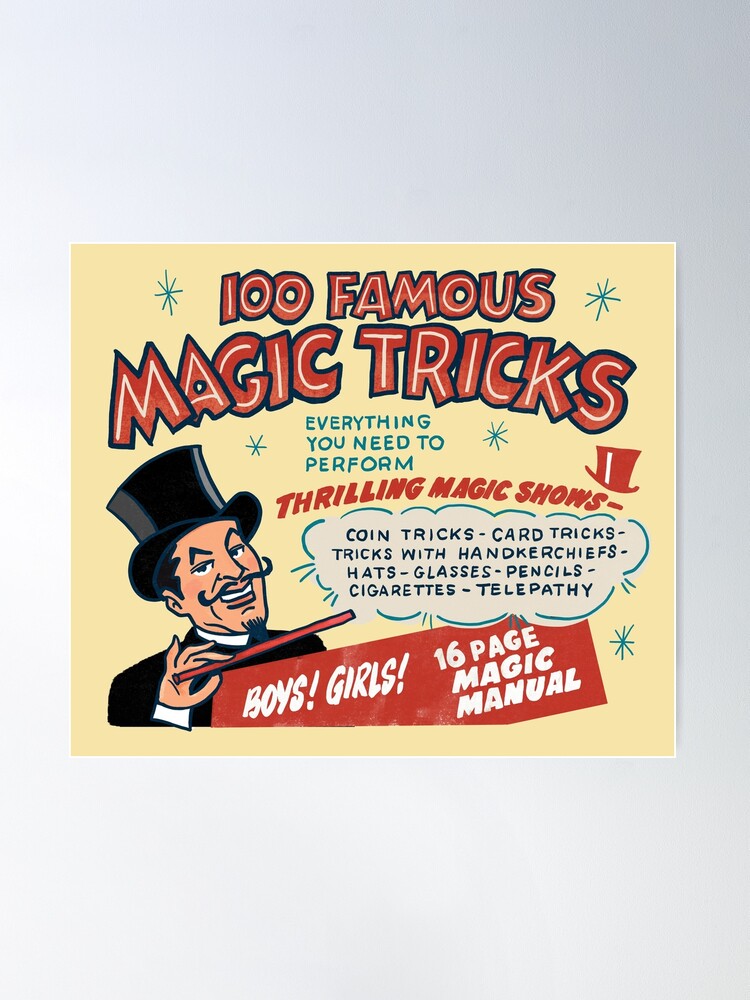This image is a detailed photograph of a small, rectangular yellow paper manual set against a white background. The top of the manual features the title "100 Famous Magic Tricks" in bold red text with a thin black outline and a yellow stripe through each letter. Flanking the title are blue asterisks. Directly below, in blue text, it reads "Everything You Need to Perform," followed by "Thrilling Magic Shows" in red. There is a whimsical white cloud with a light blue outline listing various magic tricks: "Coin Tricks," "Card Tricks," "Tricks with Handkerchiefs," "Hats," "Glasses," "Pencils," "Cigarettes," and "Telepathy." A cartoon magician adorned in a black top hat, with a curly mustache and goatee, holds a red magic wand and a red banner that declares in white text, "Boys, Girls! 16-page magic manual."